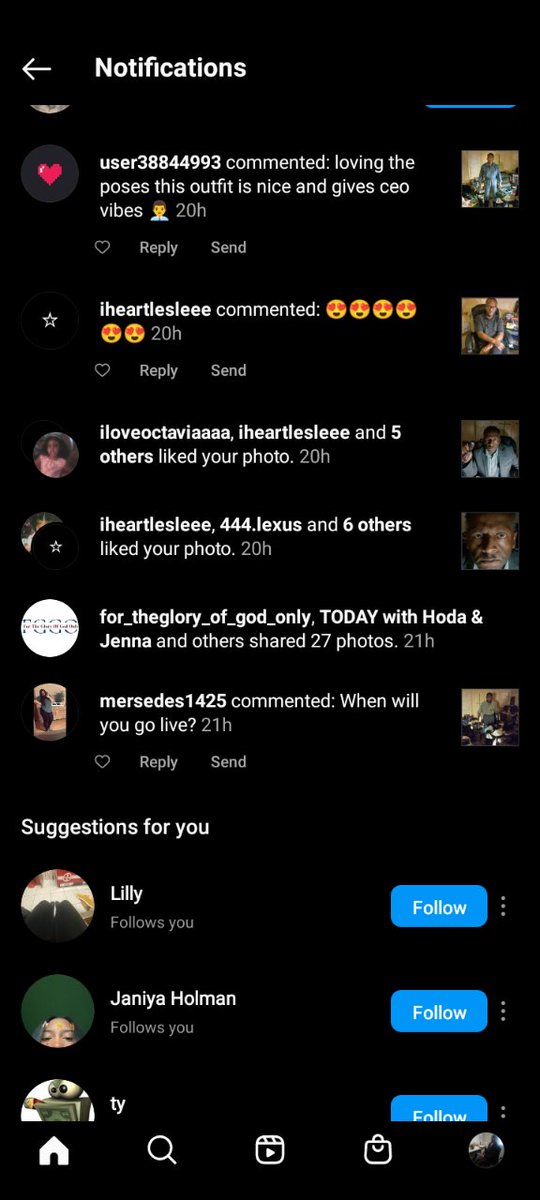The image features a sleek black background. On the left side, a white arrow points left, adjacent to the word "Notification" in bold white letters. Below this, a thin blue line runs down the right-hand edge. 

Beneath the blue line, there's a comment from user 38844993, indicated by a gray circle with a red heart in the middle. The comment reads, "Loving the poses, this outfit is nice and gives CEO vibes," timestamped 20 hours ago. To the right of this comment, a small thumbnail image is displayed.

Following that, iHeartLeslie commented with six emojis showing hearts over the eyes, also timestamped 20 hours ago, accompanied by a small star icon. Just below that, it states "I love Octavia, iHeartLeslie, and five others like your photo," again timestamped 20 hours ago. Further down, it lists "iHeartLeslie and 444.lexus and six others like your photo," at the same 20-hour mark.

The final section shares a post from "for_the_glory_of_god_only," mentioning "Today with Hoda and Jenna and others shared 27 photos."